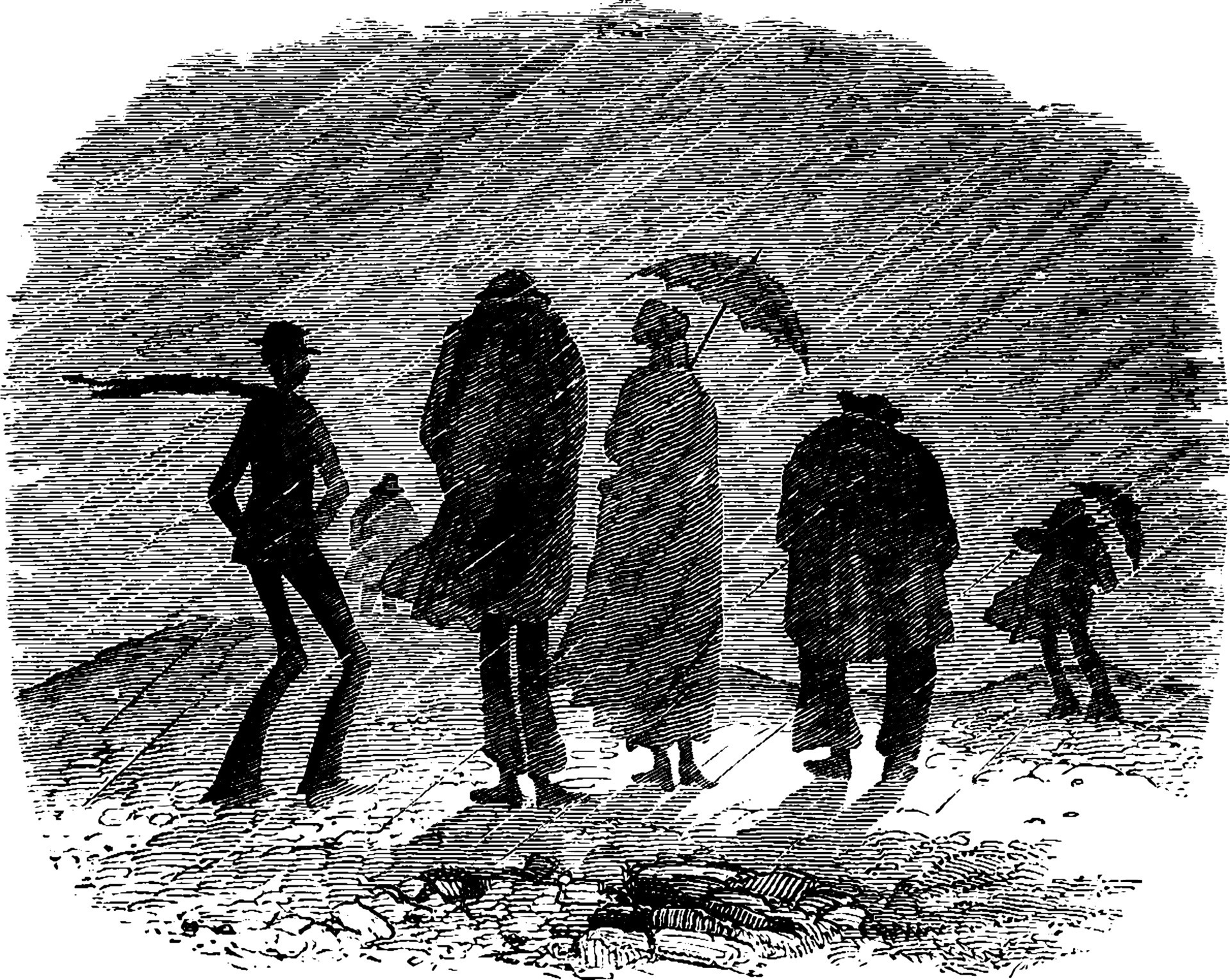This intricate black-and-white drawing, reminiscent of an etching with its detailed line work and crosshatching, portrays a scene of characters caught in a rainstorm. The entire composition is made up of textured lines that combine to create a cohesive image. Central to the scene is a woman, distinguishable by her long dress and the umbrella she holds, shielding her from the angled white lines that depict the rain. Her back, like those of the other figures, is turned toward the viewer. To her right stands a hunchbacked, portly man in a long overcoat and pants, wearing a hat. Just behind him, another tall man, also in an overcoat with a blowing scarf, appears slightly taller than the woman. At the farthest right, another figure, whose gender is indeterminate, holds an umbrella and recedes into the background. Adding to the dynamic feel of the image is a character with a cape billowing in the wind, hands in pockets, standing near the woman. Another short man with a shorter coat seems to be walking in a different direction. Together, these five distinct characters and an additional figure moving away create a vivid tableau of a windy, rainy night, all expertly rendered through the artist's masterful use of lines and texture.